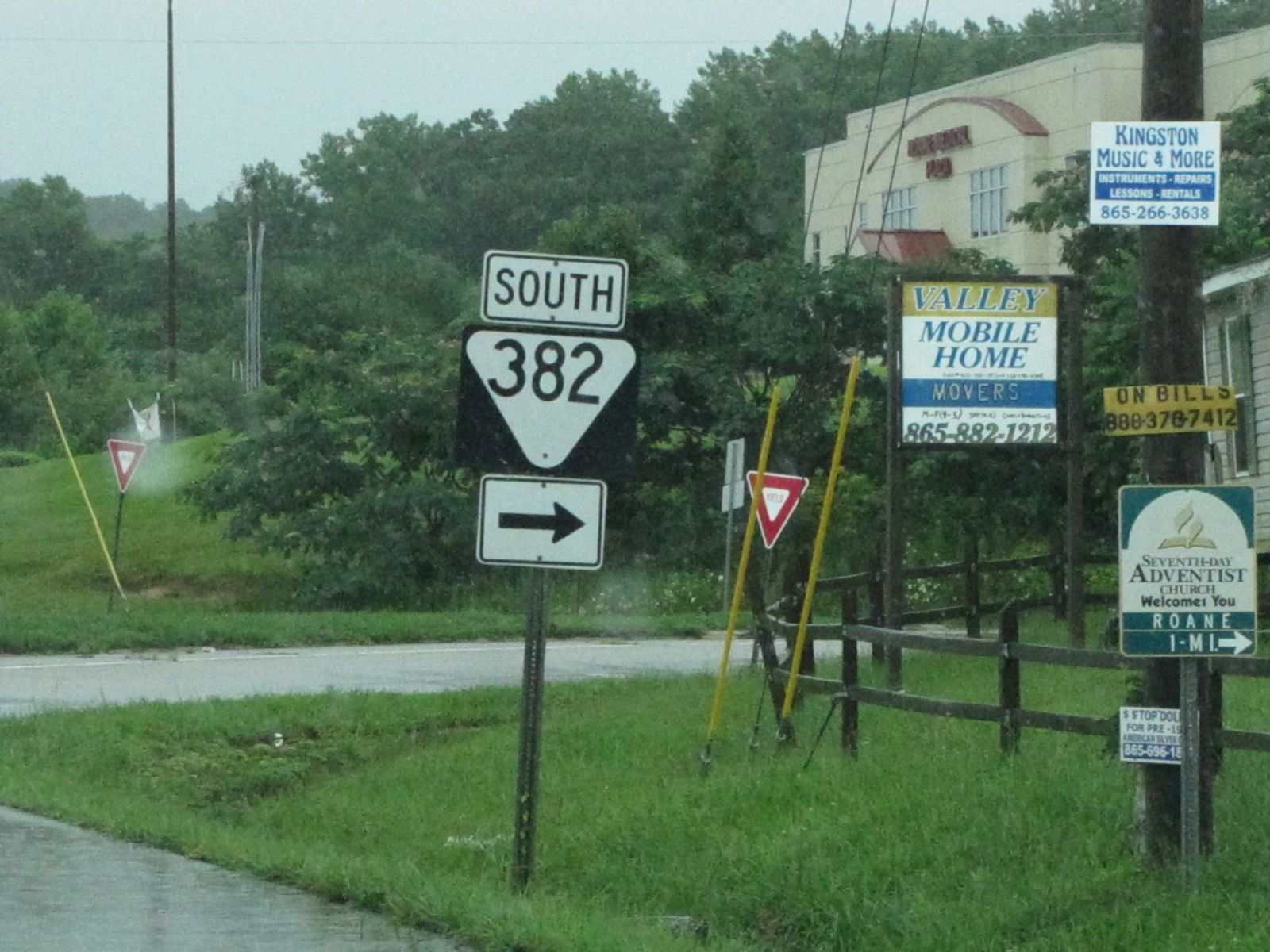In this suburban or rural scene, the image captures the corner of a road in the lower left-hand of the frame, merging into a lush grassy area that extends to the middle. Several signs dot the green field, including one prominently positioned in the center that reads "South 382" with a black arrow pointing to the left. A red yield sign adds a splash of color, while another sign nearby invites visitors to the "7th Adventist Church" one mile to the left. Additional signs advertise "Valley Mobile Home Movers," and "Kingston Music and More" along with lessons.

To the right of the South 382 sign, the scene is marked by a white triangular sign displaying the number 382 in black text against a black background with a white arrow pointing right, and a "Valley Mobile Home Movers" sign. A telephone pole, which extends out of the frame, supports the "Kingston Music and More" sign. Beyond the signs, a gently curving wooden fence and a row of green trees frame the backdrop, complemented by the overcast sky hinting at recent rain. In the distance, a tan-yellow stone office building stands amidst the greenery.

The street from which the picture is taken shows no sidewalk and merges directly into the green grass all around. Another street runs horizontally across the rear of the image, with a second yield sign positioned on the grassy area on the far side. The entire setting feels fresh and vibrant, painted with the subdued hues of an overcast sky.